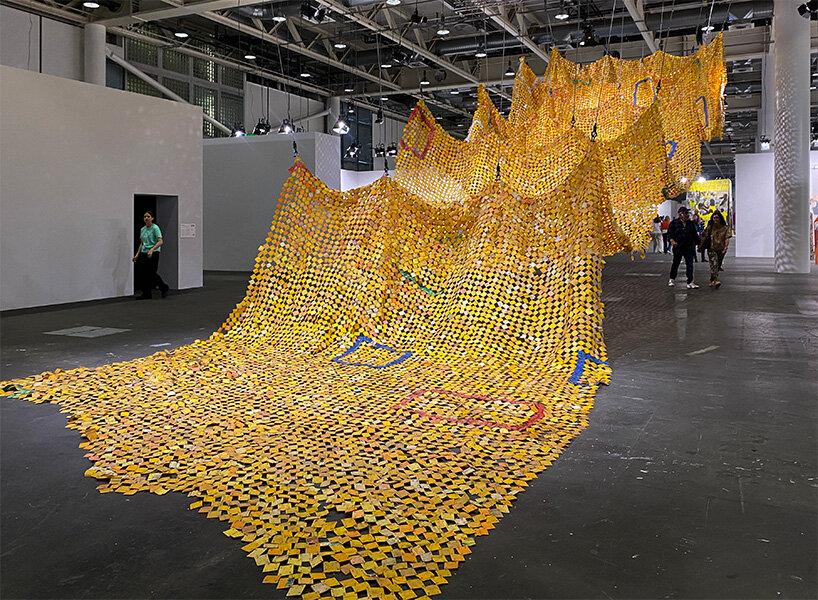The image captures an expansive, striking modern art installation in the cavernous space of a warehouse-turned-gallery, characterized by its high ceilings, crisscrossing pipes, and industrial ambiance. The centerpiece of the exhibit is a vast tapestry-like structure composed of uncountable yellow, gold, and white square pieces, reminiscent of post-it notes or small cutouts. These squares, possibly made from paper or a lightweight fabric-like material, are meticulously bonded together to form a wave-like or draping net design. Suspended by heavy-duty cables affixed to the ceiling, the installation undulates gracefully through the air, creating a rhythm of peaks and valleys before trailing onto the gray floor. Sporadically interspersed within this mass of squares are occasional pops of blue and red, adding a visual contrast to the predominantly yellow and gold hues.

In the midst of this large-scale display, several visitors can be seen: a person on the left in a green shirt and black pants, and two individuals on the right – one clad in black with white shoes and another in camouflage attire. Further in the background, a tall column ascends towards the ceiling, enhancing the sense of height and scale of the venue. Behind the onlookers, a yellow wall adorned with additional artwork serves as the backdrop, adding yet another layer to the immersive artistic experience. The soft glow from the warehouse's fluorescent lights gleams off the intricate tapestry, highlighting the craftsmanship and artistic brilliance of this elaborate installation.